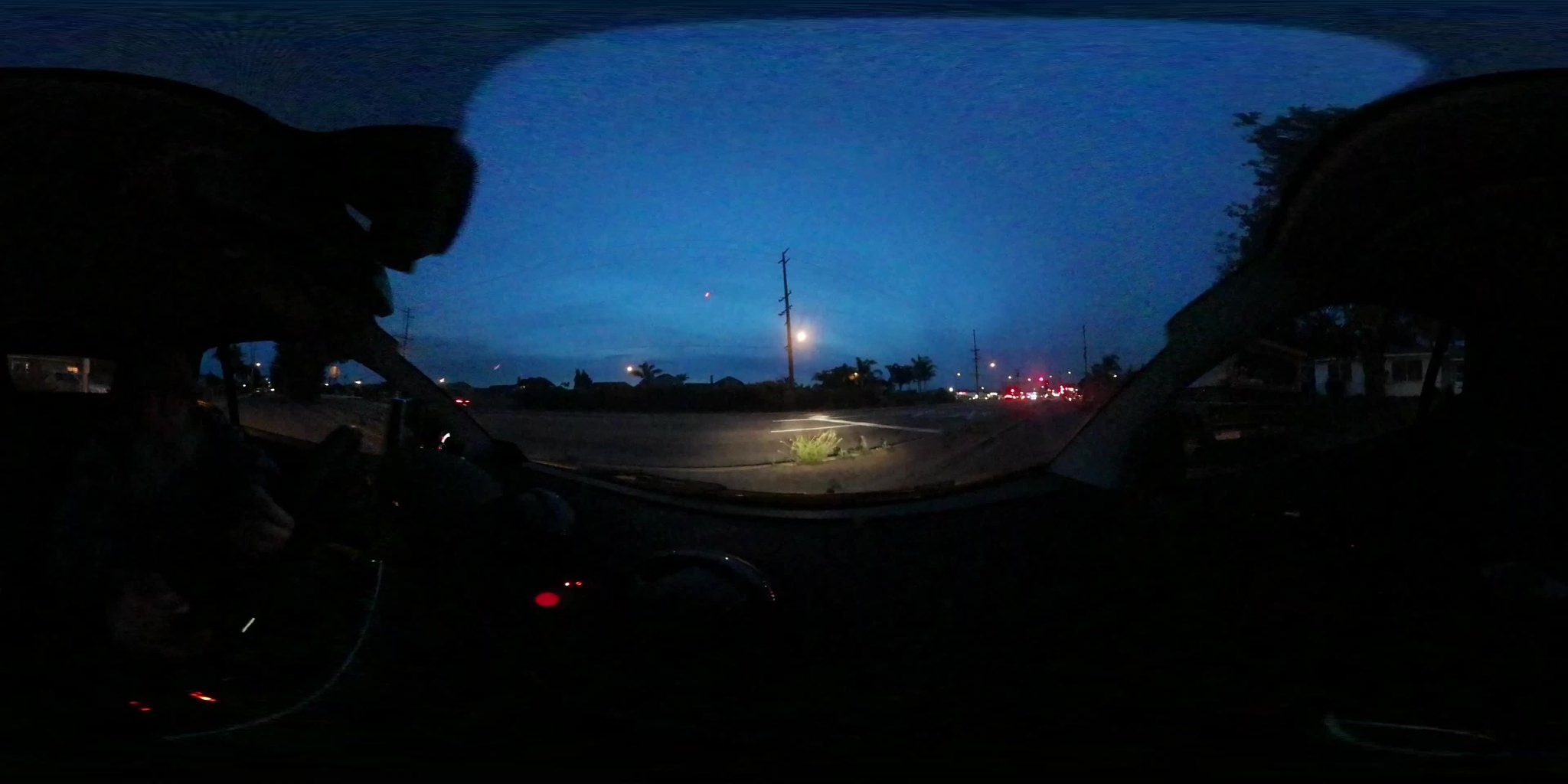A nighttime photograph possibly taken from within a car, featuring a fisheye lens effect that adds a unique distortion to the image. The scene captures a dark street, potentially at a T-intersection, under a cloudy sky lit by a small full moon. Dominating the foreground are shades of deep darkness, along with shapes resembling bushes, and the silhouette of dashboard elements from the car interior. On the left side, a lighter-colored car is partially visible, with glimpses of its taillights and passenger windows. In the distance, a series of utility poles and wires stretch out, with faint, barely discernible cables connecting them. The distant background is illuminated with many lights and perhaps even outlines of buildings, hinting at a small city or town.